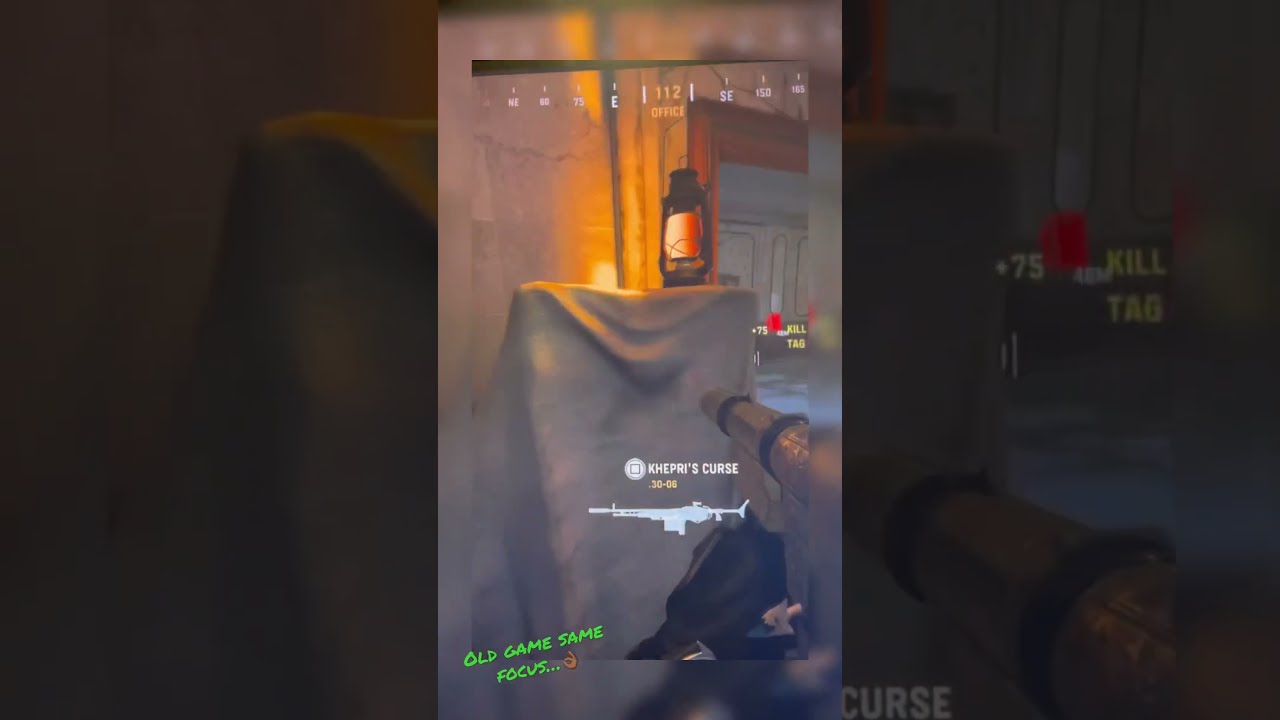In this vertically oriented, rectangular screenshot from a first-person shooter video game, the central image is clear and distinct against a faded and zoomed-in background of the same scene on either side. The player character's arms extend from the bottom edge, wielding a machine gun or rocket launcher aimed towards the center of the image. The setting appears to be an old stone warehouse with warm lamplight illuminating the walls to the left and a doorway to the right.

Centrally framed is a gray pedestal draped with a gray cloth, upon which rests an old-style oil lamp glowing orange-red. Behind the lamp, a yellow globe can be seen. White text on the pedestal reads "K-H-E-P-R-I's Curse," and just below, there is an image of a long gun. At the top of the screen, compass-like directional letters from northeast to southeast are visibly marked. In the bottom left corner, green text states "Old Game, Same Focus." Additionally, a small icon depicting a machine gun along with a video game controller button symbol is present. The detailed background images on the left and right provide an enlarged, darkened mirror of the main scene, focusing on the gun barrel on the right and the left half of the pedestal on the left.